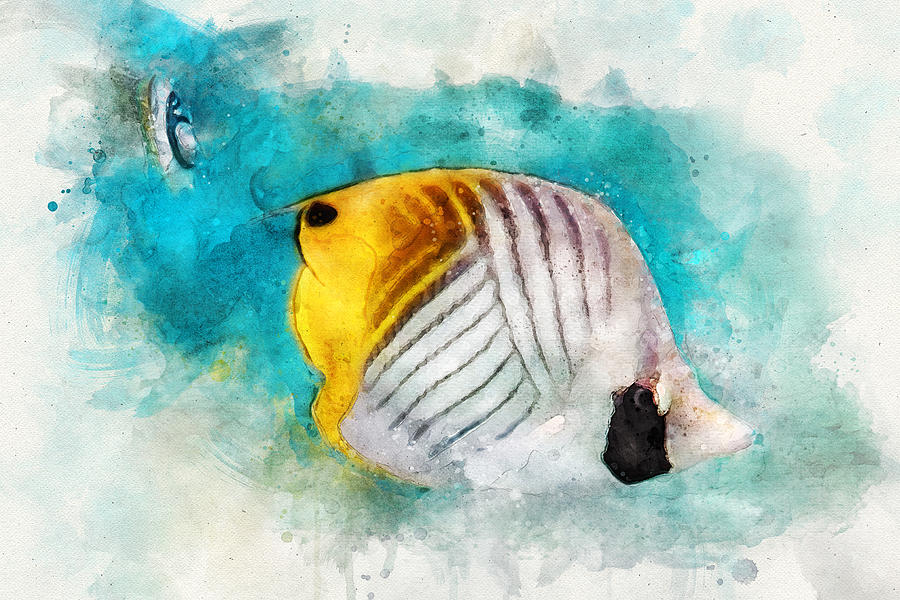This is a detailed watercolor painting set on a wide, horizontal canvas, depicting an underwater scene with vivid color transitions and a prominent fish as the main subject. The background of the painting features a blend of blues, starting with a dark blue on the left that transitions into teal and eventually a much lighter teal, interspersed with light teal water drops and flecks. The corners of the canvas are shaded in an off-white, almost light gray hue. 

In the center of the painting swims a tropical fish, viewed from the side. The fish has a rounded rectangular body shape with a pointed, white snout. Its eye is strikingly black, accompanied by a thick black stripe running horizontally from beneath the eye down to the edge of its body, creating a smudged effect. The fish's scales are fanned out in white, while the tail boasts a brilliant gold color. Midway through the body, there's a transition in the fish's coloring from a silverish white at the front to bright yellow towards the back, interspersed with brown bands and a unique lavender tint across its head. This whimsical aquatic scene is brought to life with splashes of lavender and white in the background, creating a mesmerizing blend of aquatic shades and colorful detail.